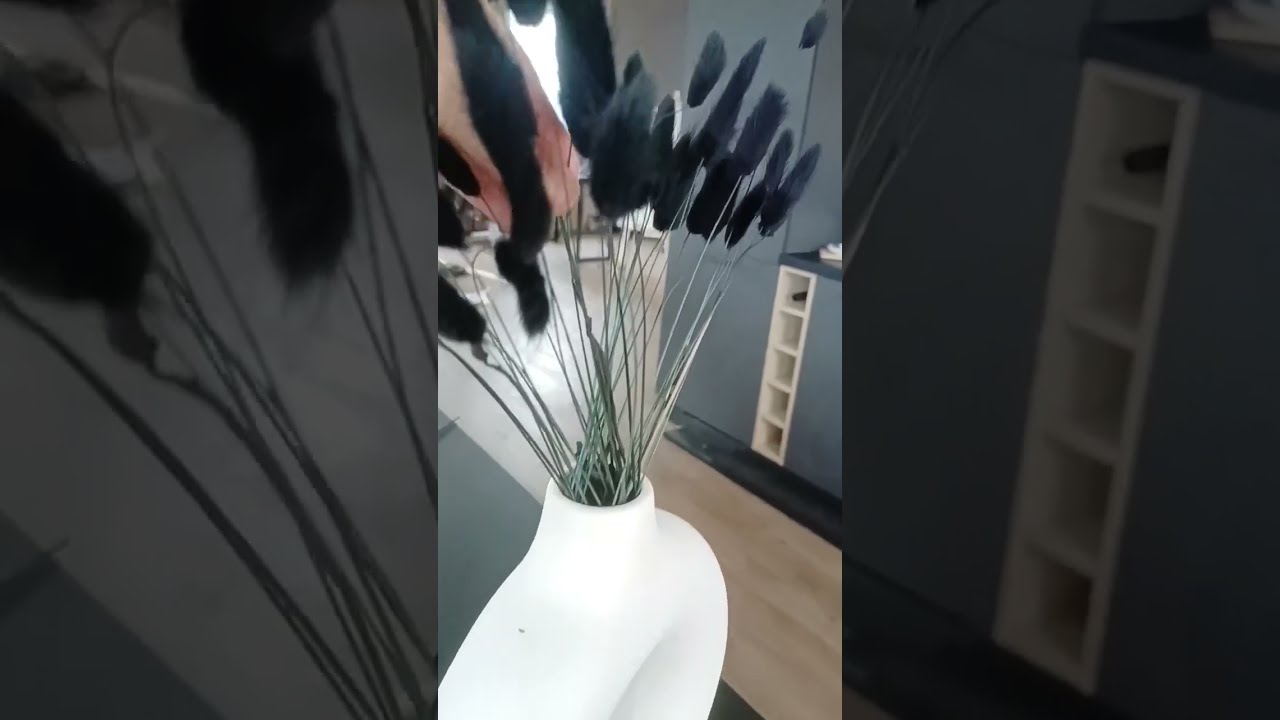In this indoor scene captured during the middle of the day, a white flower pot takes center stage, serving as the focal point of the photo. Emerging from the pot are several plants, characterized by large green stems and black-tipped flowers. The pot is situated on a wooden floor, providing a warm, natural contrast to the white container.  

In the background, we can discern built-in shelving units flanking a distant window, allowing natural light to seep into the room. The blurred effect at the edges suggests a panoramic photo, stretching the peripheral details. The image is devoid of any text and features a harmonious blend of colors including gray, white, green, black, off-white, red, orange, and yellow. This appears to be a personal home interior, thoughtfully arranged and captured through the lens.